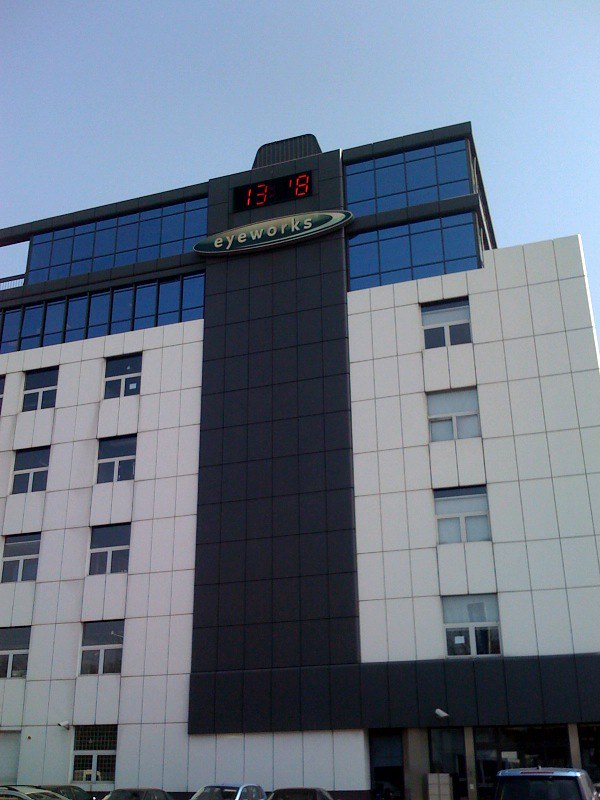The image features a towering building with seven floors. At the top, a digital display reads "13," followed by a small horizontal line and the number "8." Below this display, a sign indicates the building's name, "AyeWorks," in bold letters. The top of the building is capped with a gray roof. The upper segment includes three rows of approximately 15 blue-tinted windows each, framed by a gray metallic bar that extends horizontally across the facade. The lower portion of the building, spanning five floors, is adorned with white siding, except for a central black area adding a contrasting accent. At street level, the front doors are visible along with several parked cars, completing the urban scene.